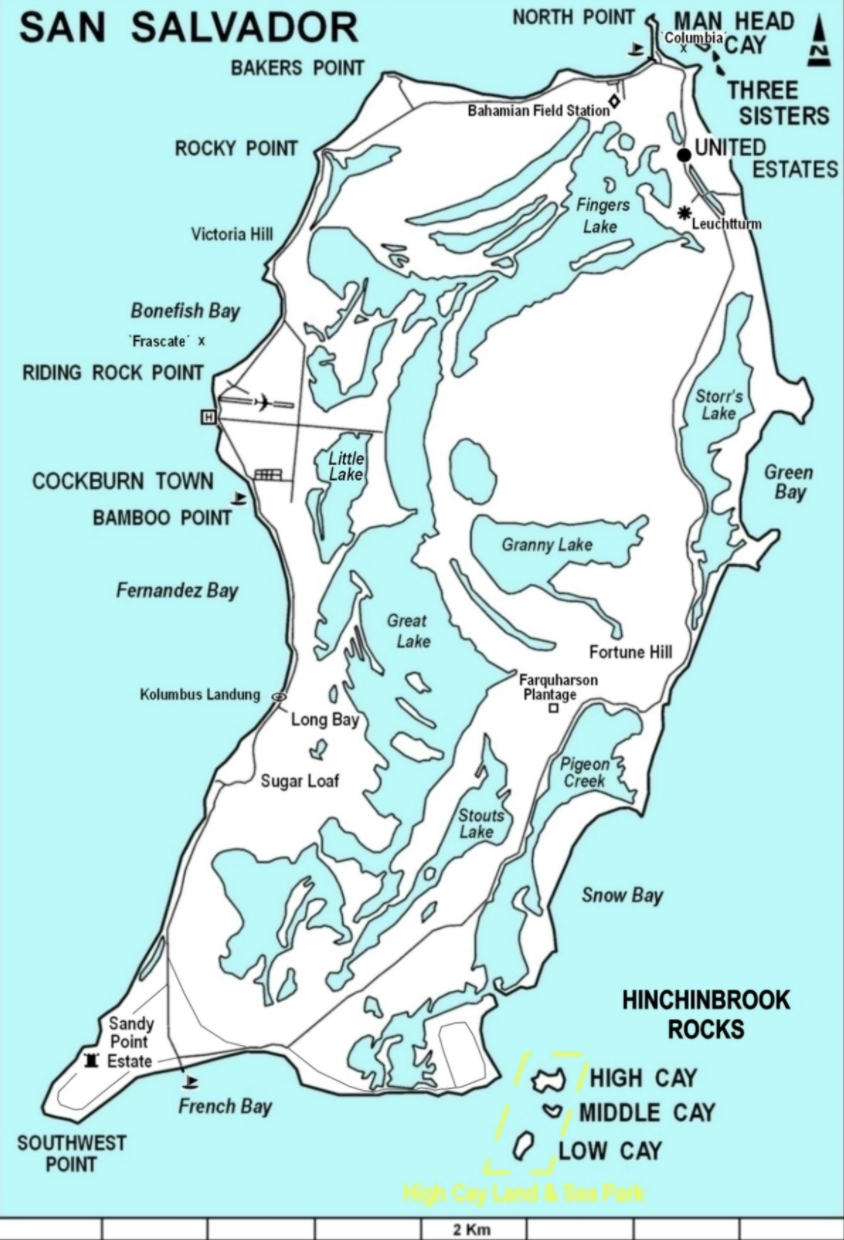This detailed map of San Salvador features a visually appealing design with a bright, light blue background that highlights the surrounding bodies of water. The island of San Salvador itself is depicted in white with clear black outlines, and the names of various locations are marked in black text. Notable points include North Point, Manhead Key, Three Sisters, Green Bay, French Bay, Fernandez Bay, Bamboo Point, Cockburn Town, Reading Rock Point, Bonefish Bay, Victoria Hill, Rocky Point, and Bakers Point. The map also identifies key lakes such as Fingers Lake, Granny Lake, Great Lake, Pigeon Lake, South Lake, and Little Lake with blue splotches. The upper left corner of the map is labeled "San Salvador" and the lower right corner reads "Hinchinbrook Rocks." The map is thoughtfully detailed, providing a comprehensive view of the island's coastal and interior geography.